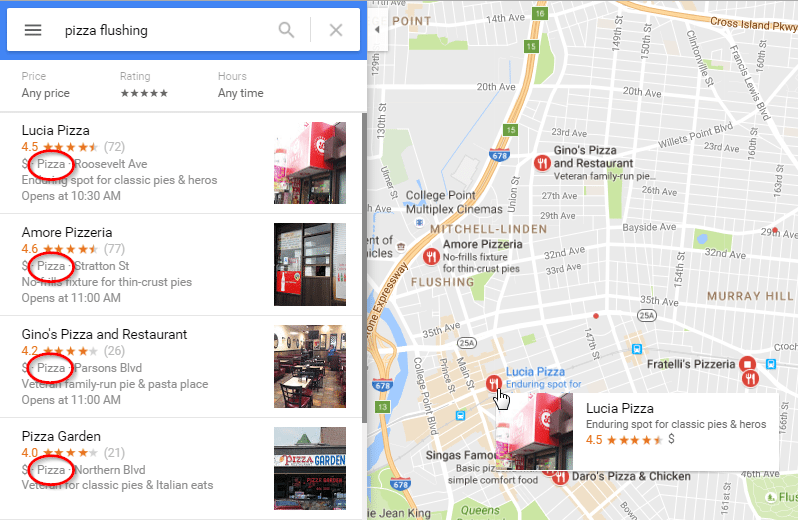The image displays a search interface specifically for finding pizza places. 

In the top-left corner, there's a search box with the query "PIZZA FLASHING." Below the search box, multiple filter options are listed: "price," "any price," "rating," "5 star rated," "hours," and "anytime." Below these filters, a list of pizza places is shown, corresponding to the search results.

1. **Local Pizza**: Rated 4.5 stars by 72 reviewers, located on Roosevelt Avenue. It offers a classic pizza experience with affordable prices and also serves heroes. The shop opens at 10 AM.
2. **Amor Pizzarella**: Rated 4.6 stars by 77 reviewers, situated on Stratton Street. It is known for its no-frills atmosphere and delicious thin-crust pies. The establishment opens at 11 AM.
3. **Gino's Pizza & Restaurant**: Rated 4.2 stars, found on Person's Belvedere. It is a family-run place offering vegetarian pies and pasta, opening at 11 AM.

**Pizza Garden** is also mentioned, located on Northern Blvd. Each pizza place name has the word "PIZZA" highlighted in red and outlined.

On the right half of the image, there is a map displaying the locations of these pizza shops. The map particularly highlights **Lucia Pizza**, which is rated 4.5 stars. The rating stars are colored orange. Additionally, images of the pizza stores are aligned on the right side, next to the map.